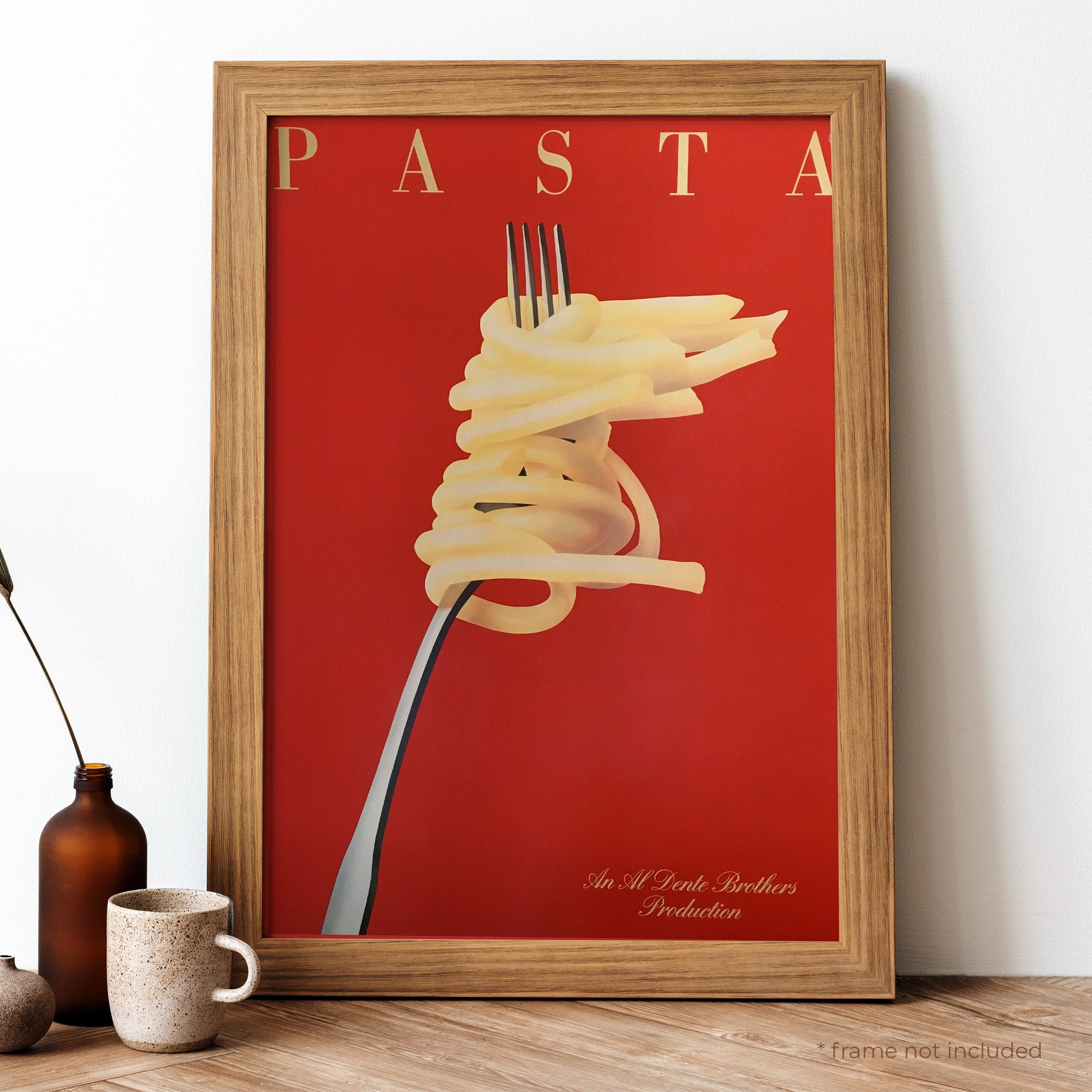The image features a vibrant red poster encased in a light blonde wooden frame, leaning against a white wall on a medium brown hardwood floor. The poster showcases the word "pasta" in distinct yellow letters at the top, and prominently displays a silver fork standing upright with spaghetti noodles intricately wrapped around its tines. In the bottom right corner, the poster is adorned with the phrase "An Al Dente Brothers Production" in elegant cursive, also in yellow. Alongside the framed poster, resting on the floor, is a beige speckled coffee mug, a brown bottle with a reed protruding from its neck, and a small, rounded black vase with a narrow opening. A note at the bottom right of the image states "*frame not included."